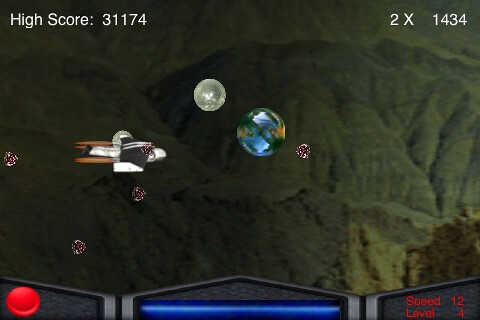This image is a color screenshot from an unidentified video game featuring a spacecraft navigating through a visually complex environment. At the top left corner, white text displays a "High Score" of 31,174, with each word’s first letters capitalized. On the top right, additional text reads "2X" beside a numerical score of 1434. The game's interface further includes a critical HUD detail on the bottom right, indicating "speed 12" and "level 4" in red text.

The background showcases a rocky, mountainous terrain or possibly a wrinkled, fabric-like surface, setting a dark, earthy tone. Prominently in the center is a large blue sphere with brownish markings, resembling an Earth-like planet or a marble. To its upper left, there is a larger, almost white opaque orb with a reflective surface reminiscent of a moon. Just below the center, a smaller speckled brown sphere adds to the celestial scene.

A white spaceship is depicted in the foreground, flying towards the right, surrounded by numerous circular objects. Among these are smaller red circles and reddish-colored spheres. A conspicuous round pearlescent orb is centrally located, adding to the detailed and immersive experience of the game.

Additionally, on the bottom left side of the screen, there is a red button resembling a control console, accompanied by a long blue line at the center, suggesting interactive gameplay elements. The meticulous composition of graphical elements provides a detailed and engaging visual representation of the space flight game.